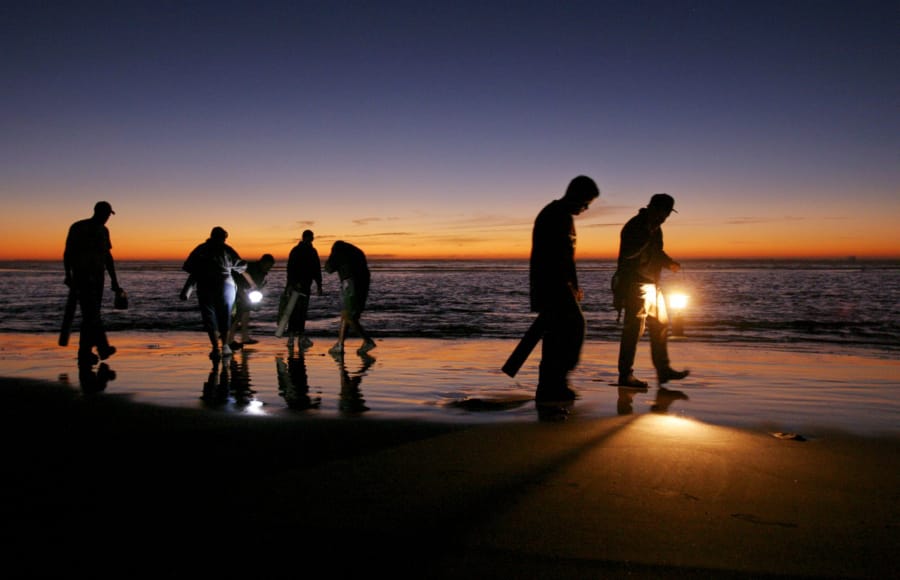The photograph captures a tranquil beach scene during twilight, with a deep, dark blue sky overhead transitioning to a vibrant orange and yellow glow at the horizon, hinting at either sunrise or sunset. The ocean waves gently lap against the shore where seven men are dispersed, five on the left and two on the right, all appearing as silhouettes against the illuminated sky. The men on the right are preoccupied, one holding a large metal cylinder and the other a bright yellow lantern, casting light onto the wet sand. On the left, the leftmost man also holds a black cylinder, while the second from the left clutches a white ball of light. These figures seem to be searching the sand, their indistinct forms underscored by the delicate interplay of light and shadow on the beach. The serene composition is complemented by the reflective sheen of the wet sand that mirrors the sky's stunning colors.